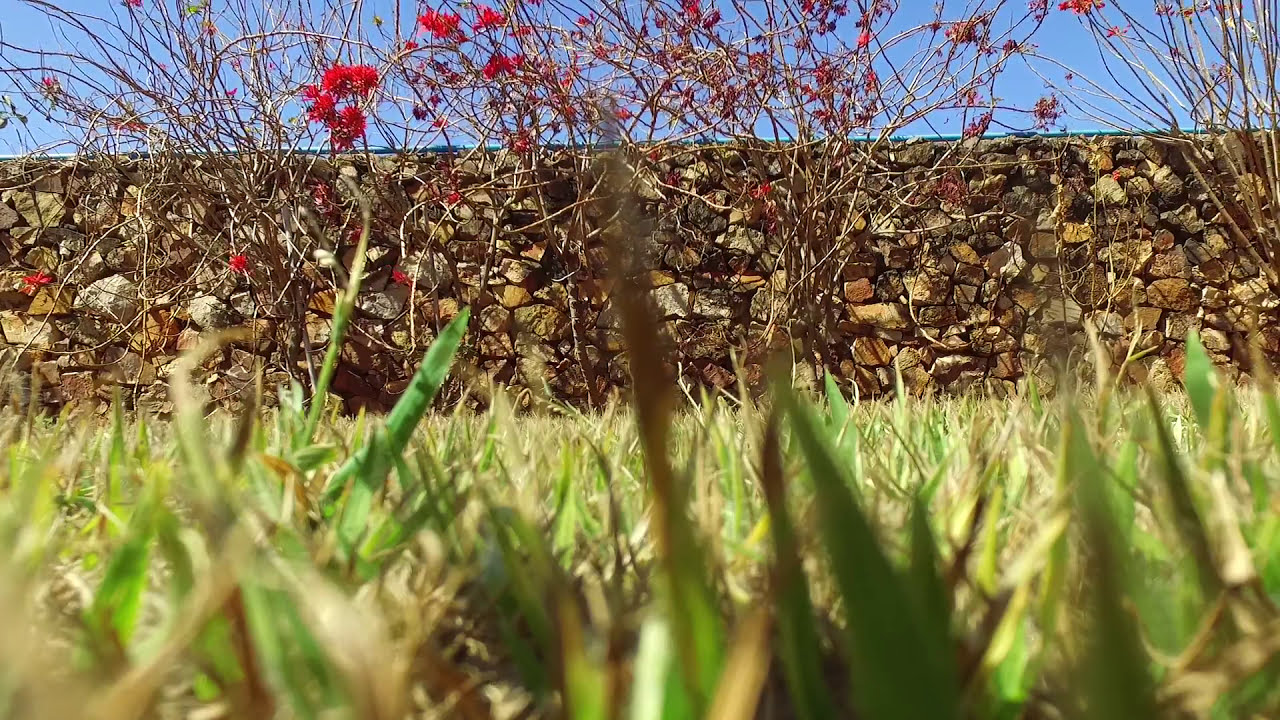This image captures a serene spring scene from a unique, ground-level perspective. In the foreground, blades of grass in various shades of green, yellow, and brown create a detailed and immersive texture, appearing slightly shadowy and blurry up close. The grass seamlessly transitions to a stone wall composed of diverse rocks in browns, blacks, and grays, adding to the textured richness of the scene. Climbing over the stone wall are vines adorned with red flowers, suggesting the vitality of early spring. Above this picturesque blend of grass and stone is a clear, brilliant blue sky, enhancing the natural beauty and tranquility of the photograph. There are no people or text, allowing the focus to remain purely on the elements of nature.